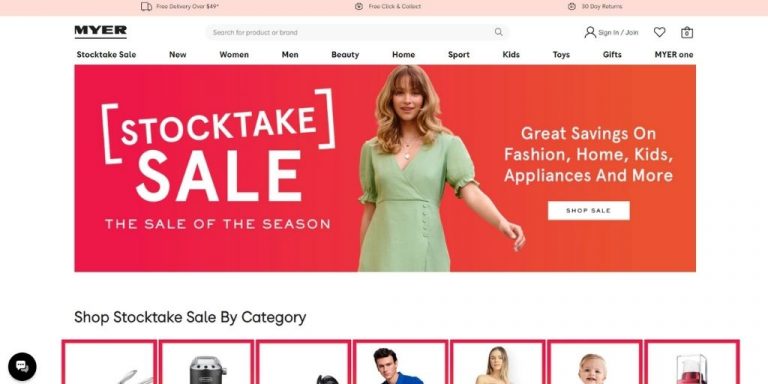This screen capture features the homepage of the Meijer website. The interface begins with a prominent pink bar at the top that contains three distinct buttons, moving from left to right: "Free Delivery Over $49," "Free Click and Collect," and "90 Days Return." Below this, the webpage's dominant white background makes the information stand out clearly. 

On the top left, there's a black, underlined "Meijer" logo. Just beneath this logo, a horizontal navigation menu lists various categories such as: "Stocktake Sale," "Meal," "Women," "Men," "Beauty," "Home," "Sport," "Kids," "Toys," "Gifts," and "Meijer One." Central to the top section is a search bar, while the top-right corner houses user interface elements including "Sign In/Join," represented by an icon of a human figure, alongside a heart icon and a camera icon.

The center of the page prominently features a large red banner with white text announcing the "Stocktake Sale, the Sale of the Season." The banner's left side shows a woman with long blonde hair, wearing a green dress, and raising her left hand, making direct eye contact with the viewer. To the right of the woman, white text highlights, "Great savings on fashion, home, kids, appliances and more." Beneath this text is a white button with "Shop Sale" in black text.

Continuing downward, a black text header reads "Shop Stocktake Sale by Category," followed by a series of seven images representing different product categories. These images include a knife, a coffee machine, the top of a black cylinder, an image of a man, a woman, a baby, and what appears to be a plastic container.